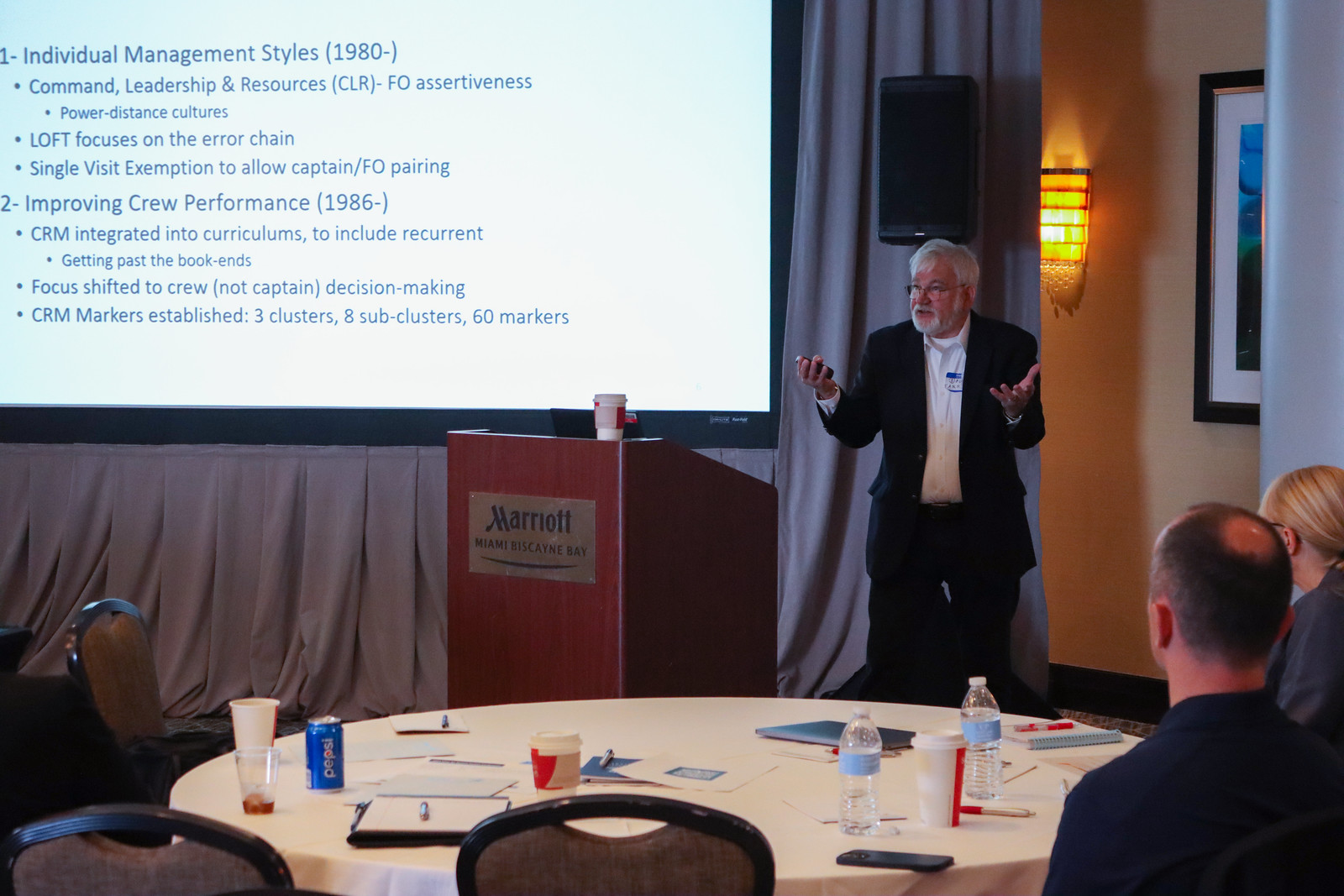The photograph captures an indoor scene at what appears to be a conference or seminar held at a Marriott Hotel, indicated by a plaque on the wooden lectern in the center of the room. In the foreground, there is a large round table cluttered with papers, writing tools, water bottles, and cups, with two people seated on its right side and several empty chairs. The focus of the image is an older man with white hair, a white beard, and glasses, dressed in a dark suit without a tie and a white shirt. He stands next to the lectern, energetically gesticulating with both hands mid-speech. He holds a clicker and appears to be discussing the contents of a slide projected on a screen behind him to the left. The slide is titled "Individual Management Styles," with detailed points about command leadership, resources management, and improving crew performance. The scene is complemented by pink curtains in the background, adding a subtle touch to the setting.